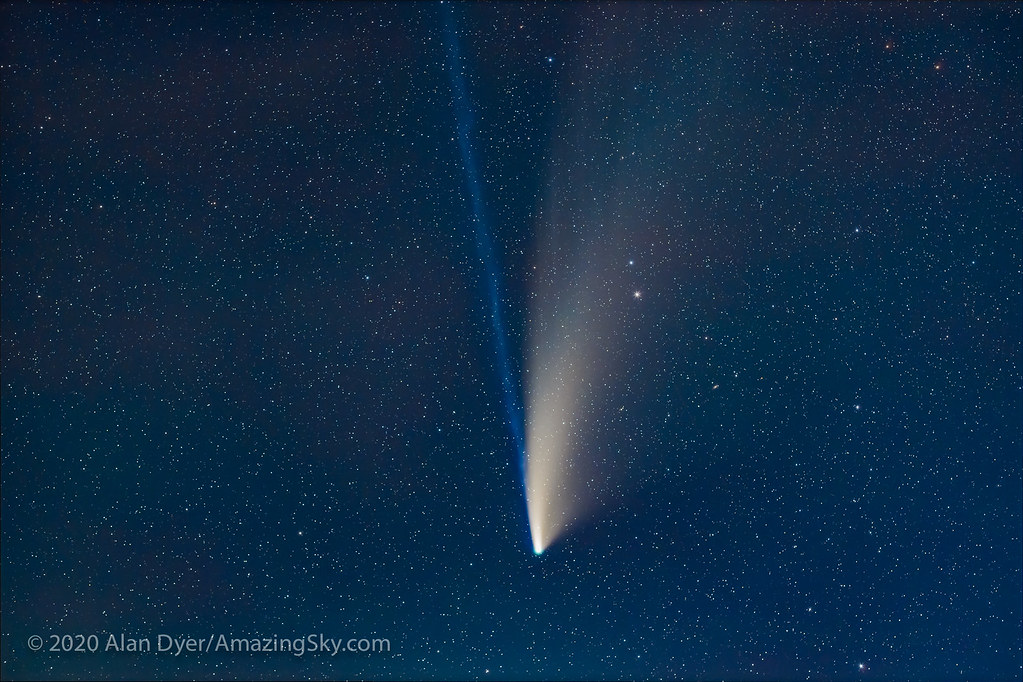This photograph, captured by Alan Dyer in 2020, showcases a breathtaking night sky filled with countless stars, depicted as tiny white dots scattered across a deep dark blue background. Dominating the scene is a bright celestial object, either a meteorite or comet, descending from the top center of the image toward the lower portion. This object leaves a striking blue trail in its wake, culminating in a radiant burst of white light in the middle of the photo, which contrasts sharply with the surrounding stars. The image is exceptionally clear, devoid of any clouds, thereby fully revealing the expansive cosmos. Notably, the bottom left corner of the photograph features a grayish-white text that reads "© 2020 Alan Dyer / AmazingSky.com," confirming the photographer's attribution. This mesmerizing capture vividly conveys the beauty and intricacies of the night sky.